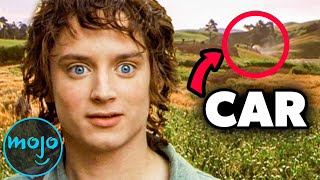The image is a close-up shot of Elijah Wood, portraying Frodo from the Lord of the Rings. His wide, pale blue eyes are fixed on the camera, and his slightly open mouth combined with unkempt light brown hair dangling over his forehead conveys a look of confusion or surprise. The actor is dressed in an olive-green collared shirt. Behind him stretches a bright, sunny landscape that could be the Shire, filled with fields and wildflowers. To the bottom right of the image, there's a WatchMojo watermark: a blue circle with "Mojo" written inside, stylized so the 'J' resembles a nose and mouth, creating a smiley face. To the right side of Frodo's head, there's bold white text that reads "CAR," accompanied by a red arrow pointing to a red-circled area in the background. This circle points to a vague white spot, suggesting the identification of a car in the background. The details hint that this may be a meme or a humorous observation highlighting a potential continuity error in the film.